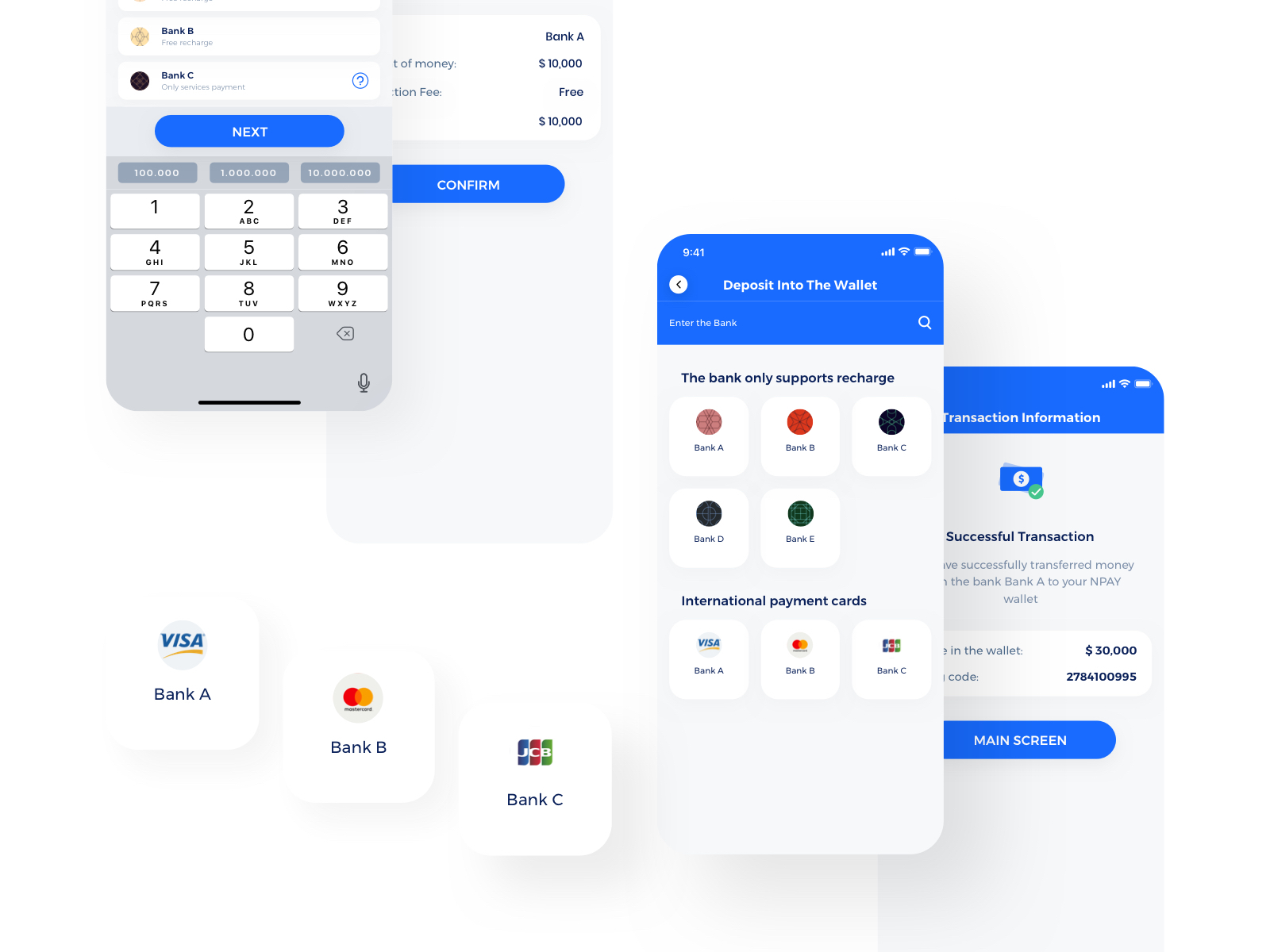The image features a detailed screenshot of a banking application interface. On the left side, icons for Bank B with a yellow circle and Bank C with a dark black and brown design are displayed. Beside them, a blue "Next" button is prominently visible. Below this section, a calculator or numeric keypad (numbers 1 through 0) is seen. Auto-populating numbers such as 100,000, 1 million, and 10 million are present, alongside a microphone button.

In the center of the interface, Bank A is highlighted, showing a balance of 10,000 with a notification of a free transaction fee. Bank A is associated with a Visa card, while Bank B uses MasterCard, and Bank C uses JCB, each accompanied by their respective logos. There is also a "Confirm" button below this information.

Moreover, the center of the screen displays an active application tab for depositing into a wallet. This tab notes that the bank only supports recharge options. Additional banks such as Bank D and Bank E are also listed, complete with their logos in varying colors: pink, red, blue, green, and black. The international payment cards supported by this application are displayed at the bottom, including icons for Visa, MasterCard, and JCB.